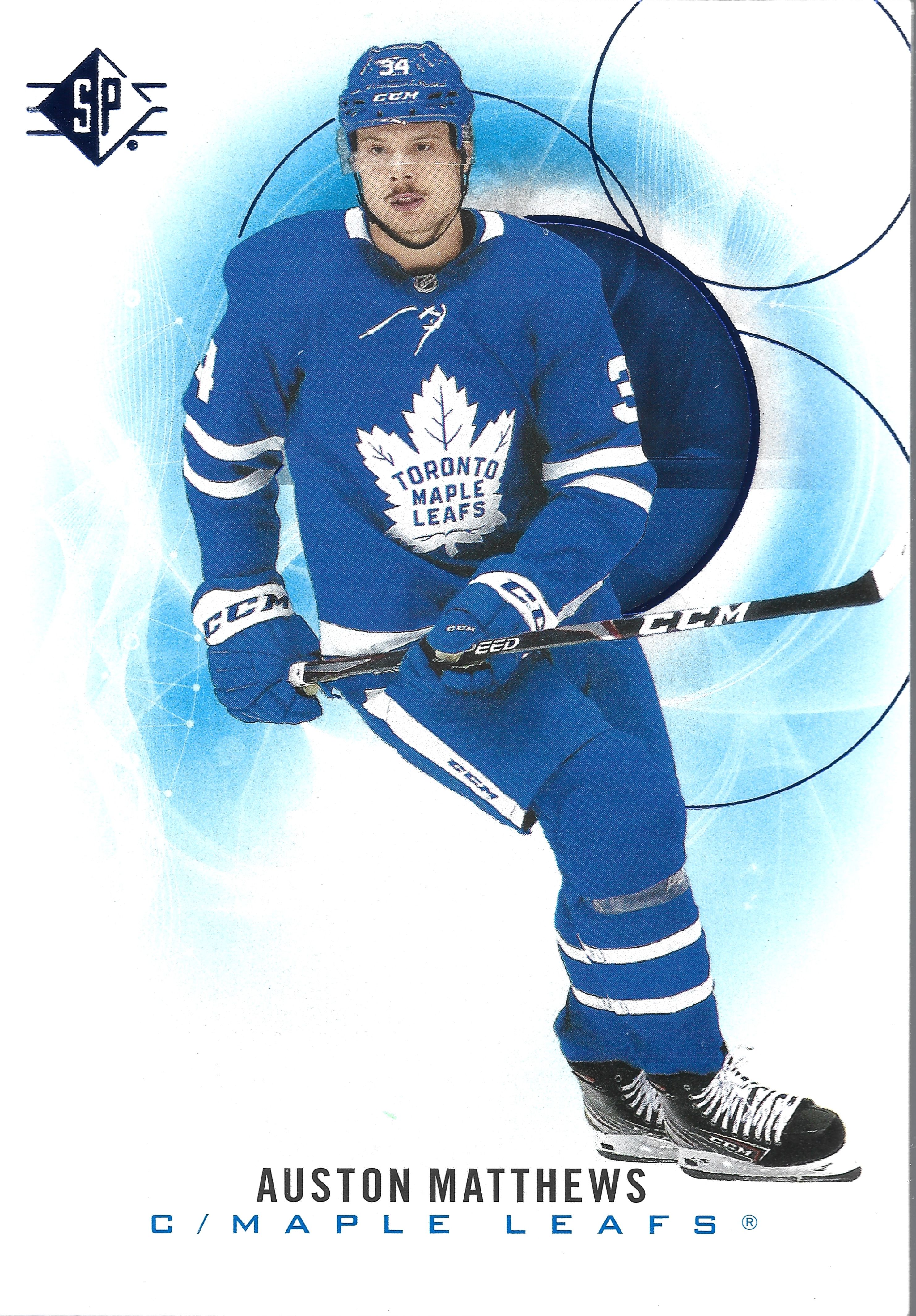This image appears to be the cover of a magazine or possibly a newspaper insert. In the top left corner, there is a logo labeled "SP." The logo is a square bisected vertically into two halves, with the left side colored black and the right side white. Behind the logo are three horizontal lines.

Dominating the cover is the main subject, a Toronto Maple Leafs player dressed in the team's iconic all-blue uniform. The team's logo, a white maple leaf with the text “Toronto Maple Leafs” inscribed on it, is prominently displayed on his jersey. The player is holding a black hockey stick and is wearing black skates.

Below the player, the text reads "Auston Matthews," followed by "See Maple Leafs" and a trademark symbol. The overall composition is both striking and informative, capturing the essence of the Toronto Maple Leafs and featuring one of their star players.